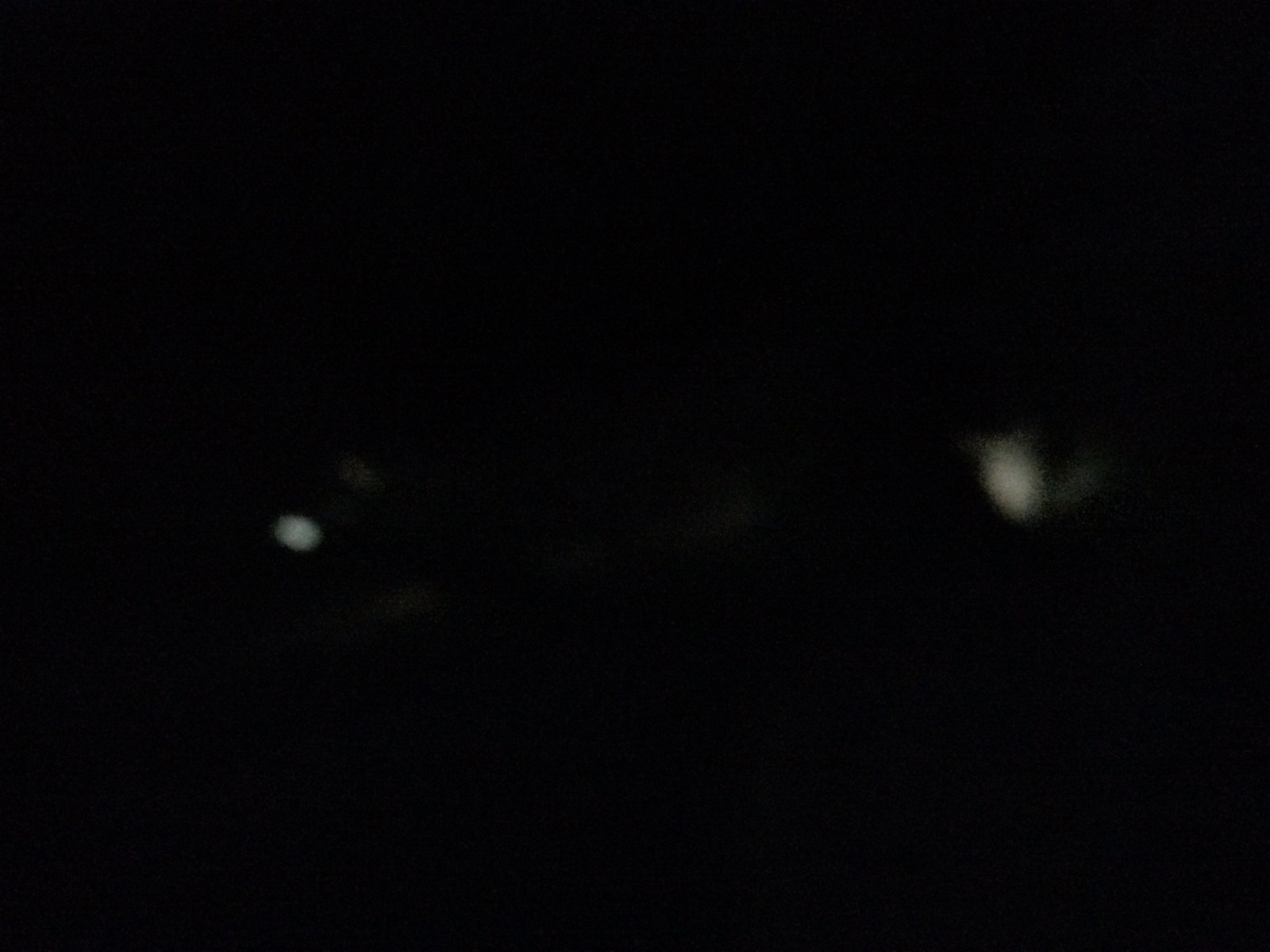This rectangular landscape photograph primarily features a solid black background with minimal contrasting elements. Positioned centrally on the left side, an unmistakable white circle stands out amidst the darkness. Adjacent to this circle, a few faint, grayish spots subtly emerge, adding texture to the scene. Beneath this collection and stretching towards the top right corner, a singular gray line traces a gentle path, connecting the composition. Shifting focus to the center-right, a distinct white oval captures attention, with a neighboring gray oval located slightly to its right and bottom, creating a balanced interplay of light and shadow against the dark canvas.